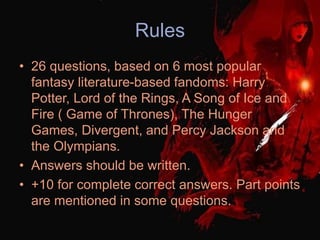The image is a square-shaped illustration that appears to depict rules for a trivia-style contest or game. The background is predominantly black with a dark red hue and a detailed, red, dragon-like figure emerging from the right-hand side. At the top of the image, the word "Rules" is displayed in blue text. Below this header, the rules are outlined in three distinct notes:

1. "26 questions based on six popular fantasy literature fandoms: Harry Potter, Lord of the Rings, A Song of Ice and Fire (Game of Thrones), The Hunger Games, Divergent, and Percy Jackson and the Olympians."
2. "Answers should be written."
3. "Plus 10 for complete correct answers. Part points are mentioned in some questions."

Additionally, there is a hooded figure with black lips located in the top right corner, seamlessly blending with the red dragon. This figure adds a dark and mysterious aura to the illustration, complementing the black background and contributing to the overall fantasy theme.